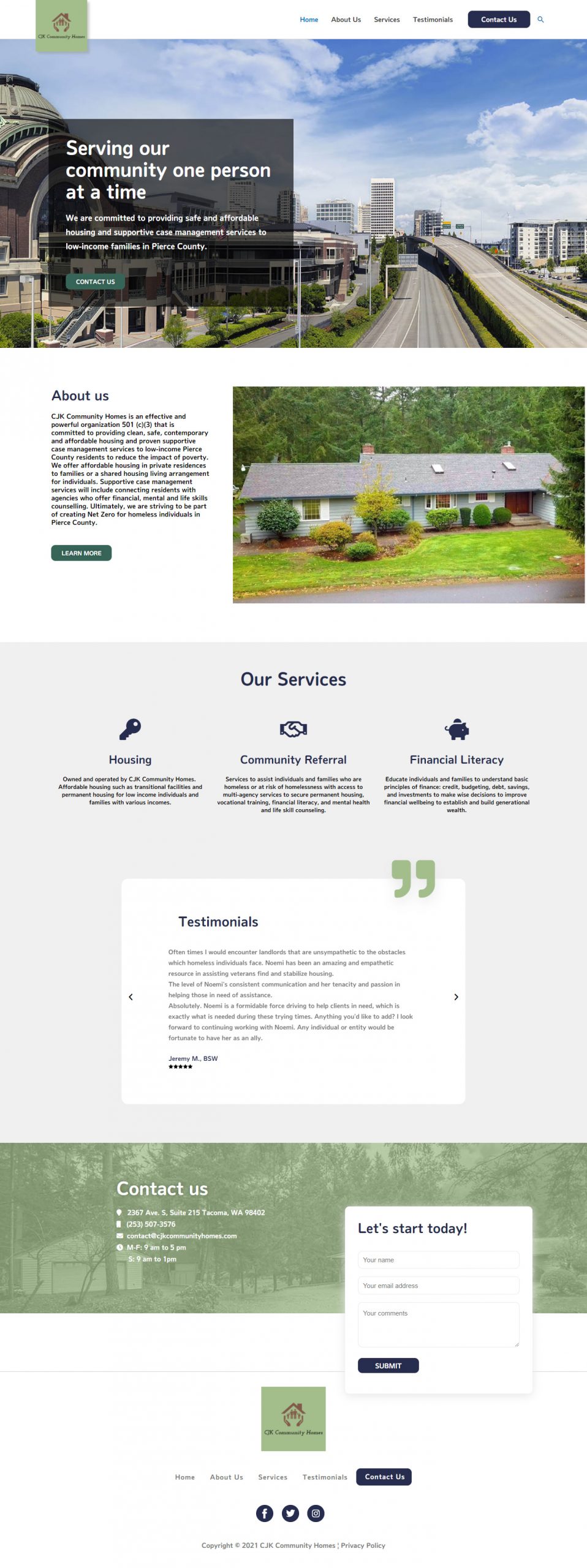"Serving Our Community, One Person at a Time"

This brochure highlights the CJK Community Homes, a dedicated 501(c)(3) organization based in Tacoma, Washington. The background features a bustling cityscape with numerous skyscrapers and business office buildings, interconnected by multiple highways.

CJK Community Homes is committed to providing clean, safe, contemporary, and affordable housing along with proven supportive case management services to low-income families in Pierce County. The organization strives to reduce the impact of poverty by offering different housing options: private residences for families and shared living arrangements for individuals.

Supportive case management services offered by CJK Community Homes connect residents with various agencies that provide financial, mental, and life skill counseling. By integrating these services, the organization aims to achieve a net-zero rate for homeless individuals in Pierce County.

Key services highlighted include:
- Housing
- Community referral
- Financial literacy

For more information and to join this impactful initiative, contact CJK Community Homes in Tacoma, Washington.

A commendable effort towards fostering a supportive and thriving community!